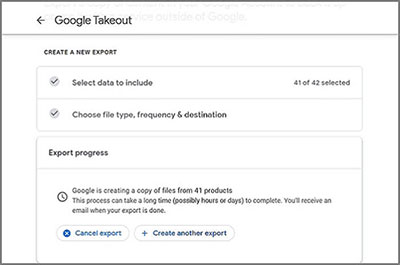**Screenshot Detailing Google Takeout Export Process**

The image displays a screenshot from Google Takeout, illustrating the export process in detail. The screen is predominantly white with black text, maintaining a simplistic and straightforward appearance. Key elements depicted include:

- **Create New Export**: A section where users initiate a new data export.
- **Select Date Range**: An option allowing users to choose the dates for which they want to include data in the export.
- **41 of 42 Selected**: Indicates that 41 out of 42 available data categories have been selected for export.
- **Choose File Type, Frequency, and Destination**: Options enabling users to specify the format of the files, the frequency of the exports, and the destination to which the exported data will be sent.
- **Export Progress**: A section that will display the progress of the data export once it begins.
- **Create Export Button**: A prominent blue button at the bottom of the screen that users click to commence the export process.

The image content remains monochromatic, featuring a white background with black text that ensures clarity and readability.